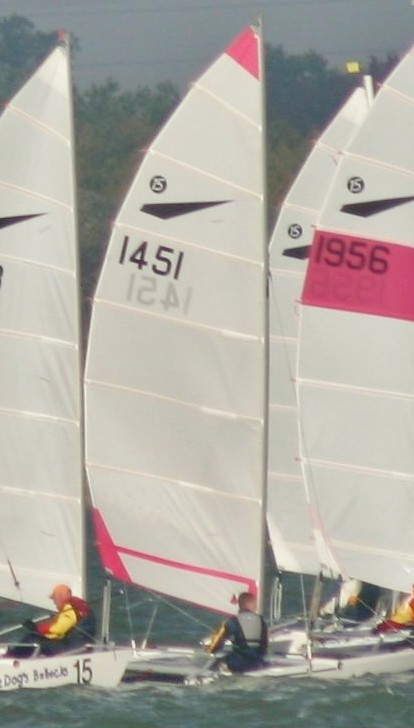This is a muted, low-resolution color photograph in portrait orientation, depicting four small sailing boats closely lined up in a row amidst rough, grayish waters. The sea and sky blend together in a similarly dull gray hue with some clouds. Each boat features tall, white sails; however, the far edges of the leftmost and rightmost sails are not visible, with the sails on the right side appearing to overlap, suggesting a fourth boat behind the visible three. The sails have white lines crossing them and are marked with numbers: the center sail displays the number 1451 above a pink triangle, while the rightmost sail has the number 1956 on a pink block. There are four individuals discernible on the boats. The person on the left wears a red jacket with yellow sleeves, and the one on the right wears a grey-blue jacket and trousers. The details of the other individuals are more obscure, though one appears to wear a white top and another a yellow and red top. The middle sail also features a logo resembling an Adidas symbol.